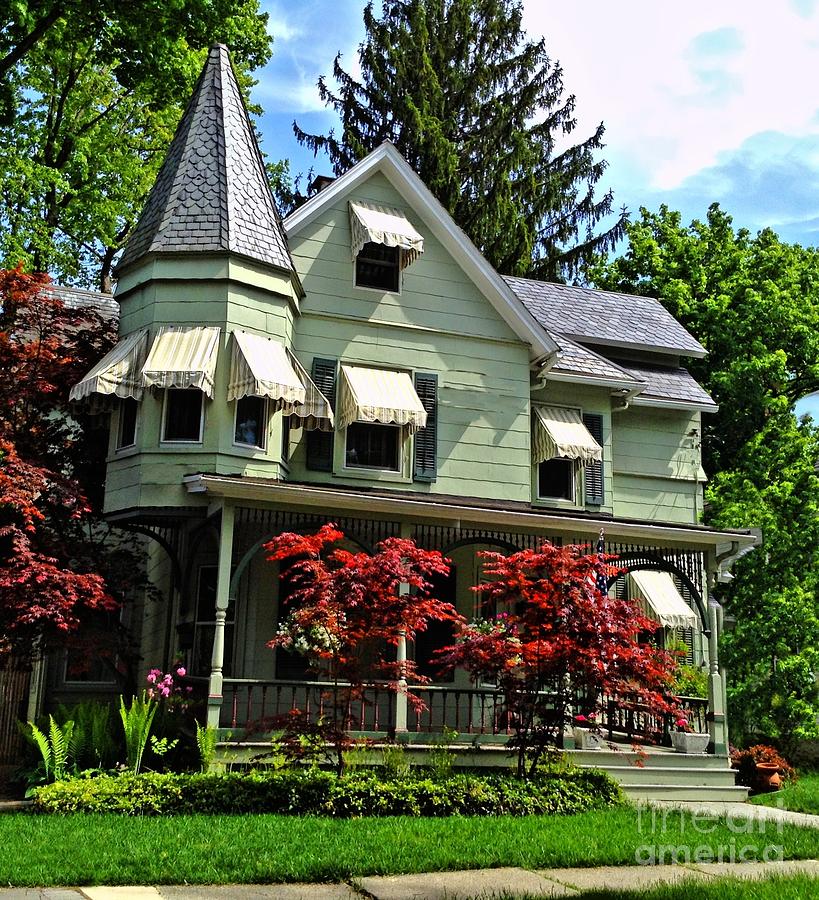This photograph captures a picturesque, Victorian-style house set against a backdrop of a clear autumn day. The three-story home, adorned with pale seafoam green siding and gray shingles, features striking architectural details such as multiple gable roofs, a turret with three windows, and various awnings over the windows, some of which are striped. The large front porch, supported by four pillars and accessed by an arch and steps on the left, stretches across the front and is complemented by what appears to be iron-wrought or dark wooden railing. In front of the porch, small red-leaf trees and vibrant green grass enhance the seasonal feel, with additional tulips and a hint of a sidewalk adding to the charm. Numerous trees surround the house, including a prominent large tree in the center back, and another significant tree to the right, each contributing to the picturesque fall ambiance. The sky is a stunning blend of blue and white, providing a serene backdrop. A Fine Art America watermark is visible in the lower left corner of the image. Despite its aged allure, the house appears to need some tender loving care, hinting at its long-standing history.